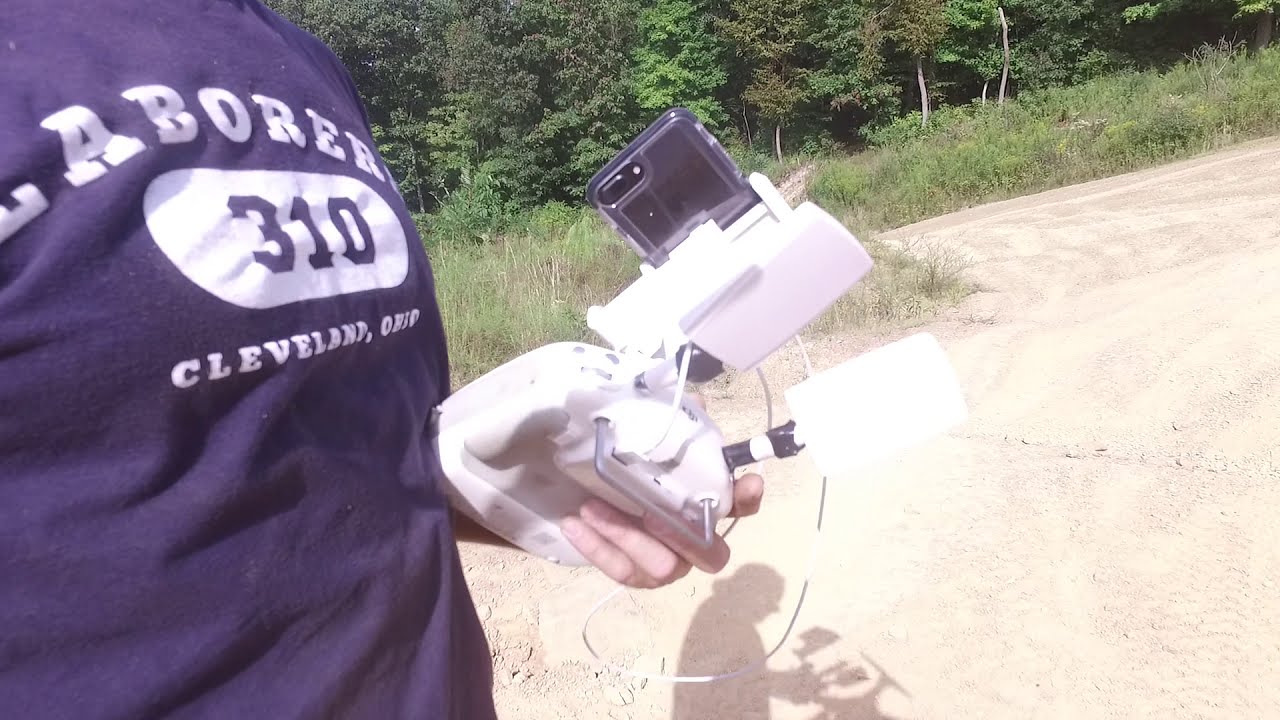This landscape-oriented color photograph captures a scene set outdoors, featuring a person standing on the left side of the image. The photograph shows the person's chest area adorned with a navy t-shirt that bears the inscription "Laborer 310 Cleveland, Ohio" in white lettering, with the number 310 displayed within a white oval background. The person's left hand, covered by a white glove, holds a device that seems to be a controller for a drone. A black attachment, possibly a holder for a smartphone or a video recorder, is connected to the top of the controller, with a cord linking the phone to the device. The shadow of the person holding the device, along with a larger drone-like object, is visible at the center bottom of the image. The backdrop features a dirt or gravel path flanked by a row of grass, extending towards a dense thicket of green trees. The scene is rendered in a photographic realism style, offering a detailed and representational depiction of the moment.